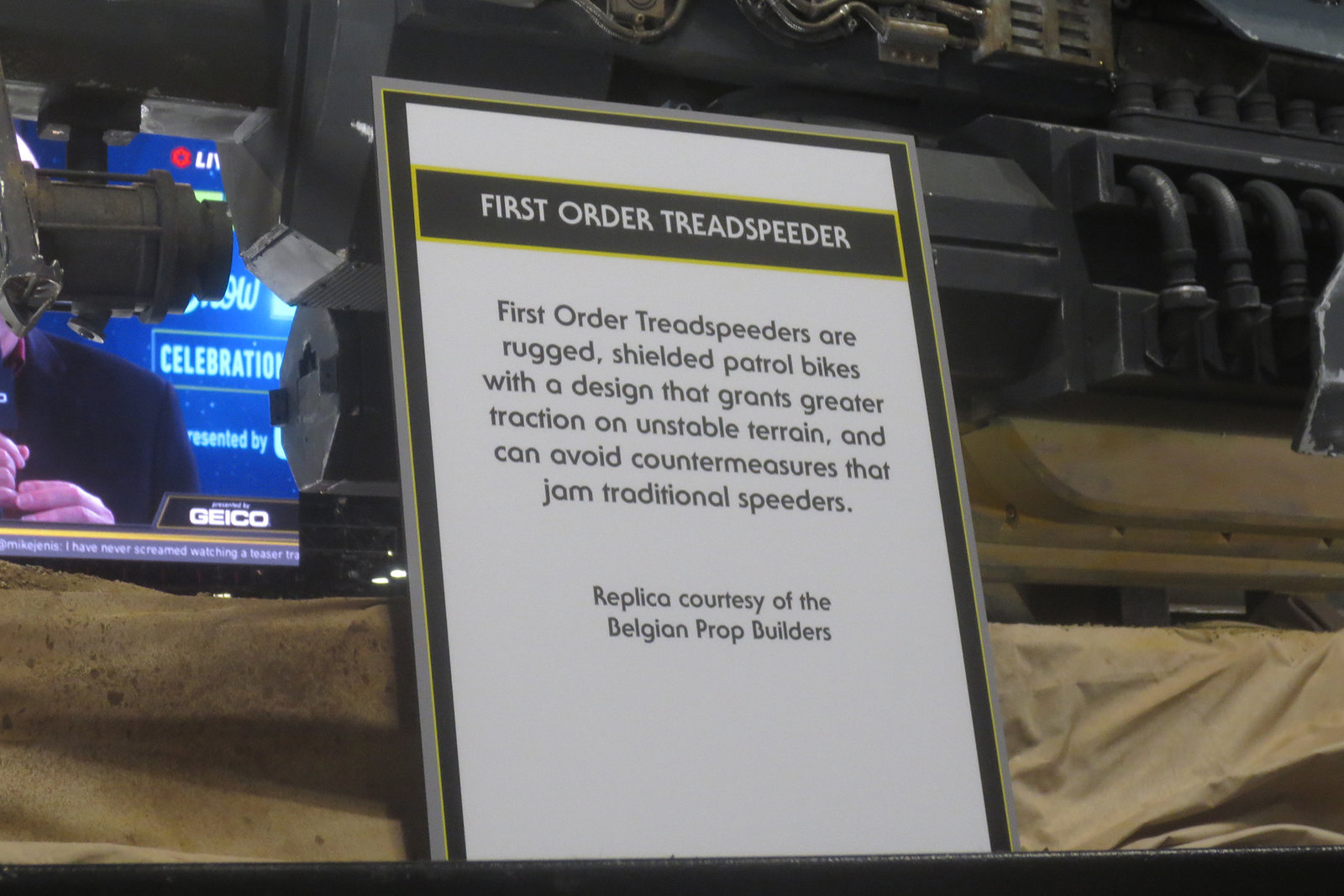The image features a detailed display sign for a "First Order Treadspeeder." The sign is framed with a silver border and contains a white inner background set against a dark brown exterior. A yellow outline highlights the text. The top section of the sign displays "First Order Treadspeeder" in bold white letters against a brown band. Below, the description reads: "First Order Treadspeeders are rugged, shielded patrol bikes with a design that grants greater traction on unstable terrain and can avoid countermeasures that jam traditional speeders." There is an acknowledgment that the replica is courtesy of the Belgian Prop Builders. The sign is placed in front of a dark, industrial-looking machine with visible pipes, possibly set against metal backdrops. Additionally, smaller text or elements like "GEICO" and "Celebration" are part of the display, seen in bright blue colors amidst the metallic surroundings.